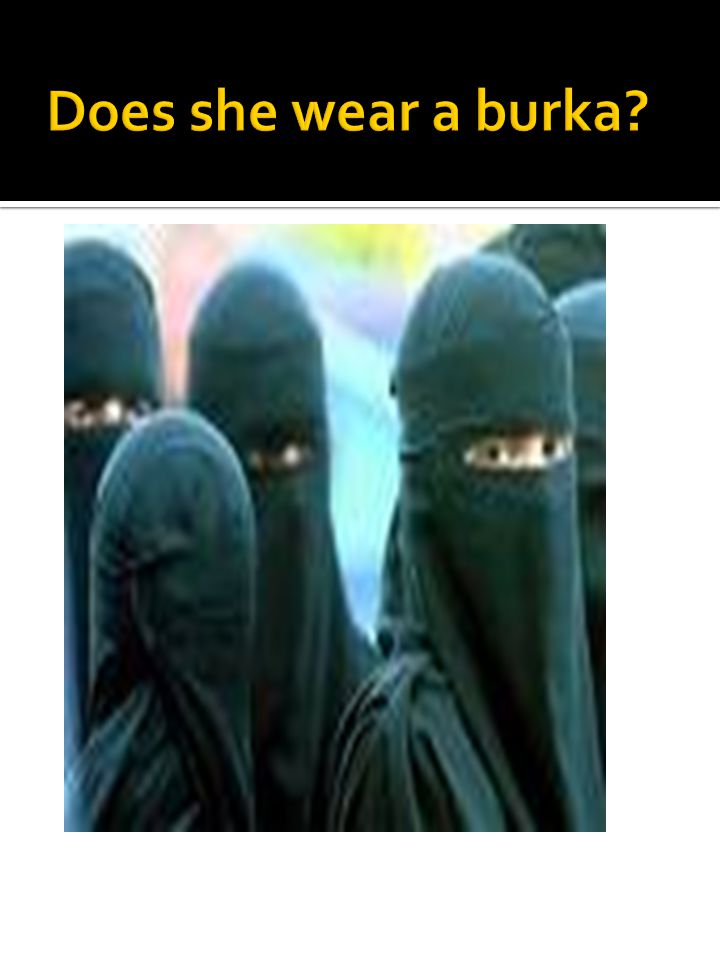The image is a low-resolution, somewhat unconventional meme. At the very top, a black rectangle spans the width of the frame, overlaid with the question "Does she wear a burka?" in bold yellow sans-serif font. Below this is a thin gray line separating the text from the main image. The main image features a group of six Middle Eastern women dressed in dark robes and headdresses that cover everything except their eyes and the bridge of their noses. 

The women are positioned against a background of pastel colors that blend in shades of light blue, pink, purple, yellow, and white, adding a somewhat abstract and fuzzy appearance. In the foreground, on the left, one woman stands with her back to the camera, making it hard to determine if her head is turned or if the eye opening of her burka is sewn shut. To the right, one woman looks directly at the camera, flanked by two partially visible women behind her. The eyes of the women are varied in expression; two have very dark eyes, and one appears to have a reddish mark near her eye, adding a peculiar detail. The overall effect is somewhat eerie and enigmatic, raising more questions than it answers.